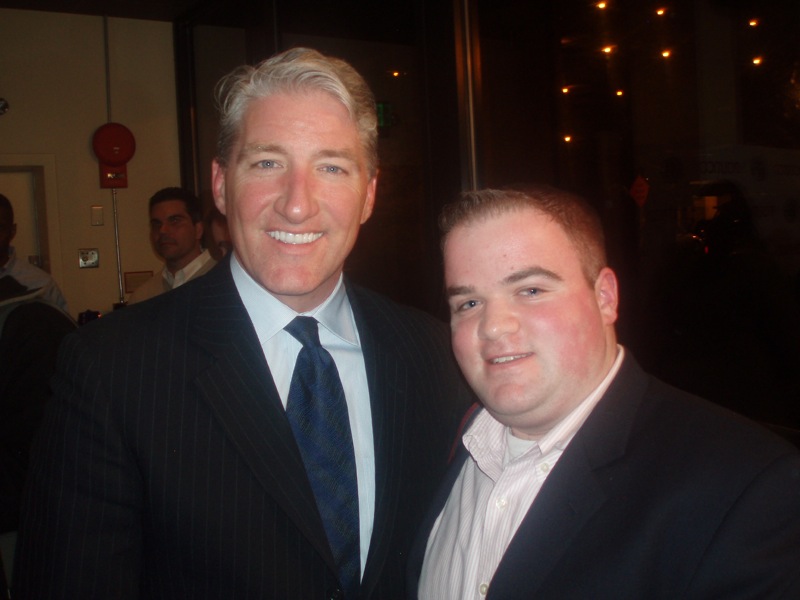This photograph captures two white men standing together at an event, likely a meeting or convention. The man on the left, an older gentleman in his 50s with gray hair and blue eyes, is recognized as a CNN host known for his election breakdowns. He is dressed in a pinstripe black suit jacket, a white shirt, and a blue tie, and he is smiling, revealing very straight and white teeth. The man on the right is a bit shorter, seemingly in his 20s, with shorter brown hair and rosy cheeks. He is wearing a black suit jacket and a white button-down shirt and is also smiling slightly. In the background, other people can be seen towards the left, along with the cream-colored walls and a glass window that reflects the room but appears mostly dark. Some lights and a structure that appears to be a stage are visible on the right side.